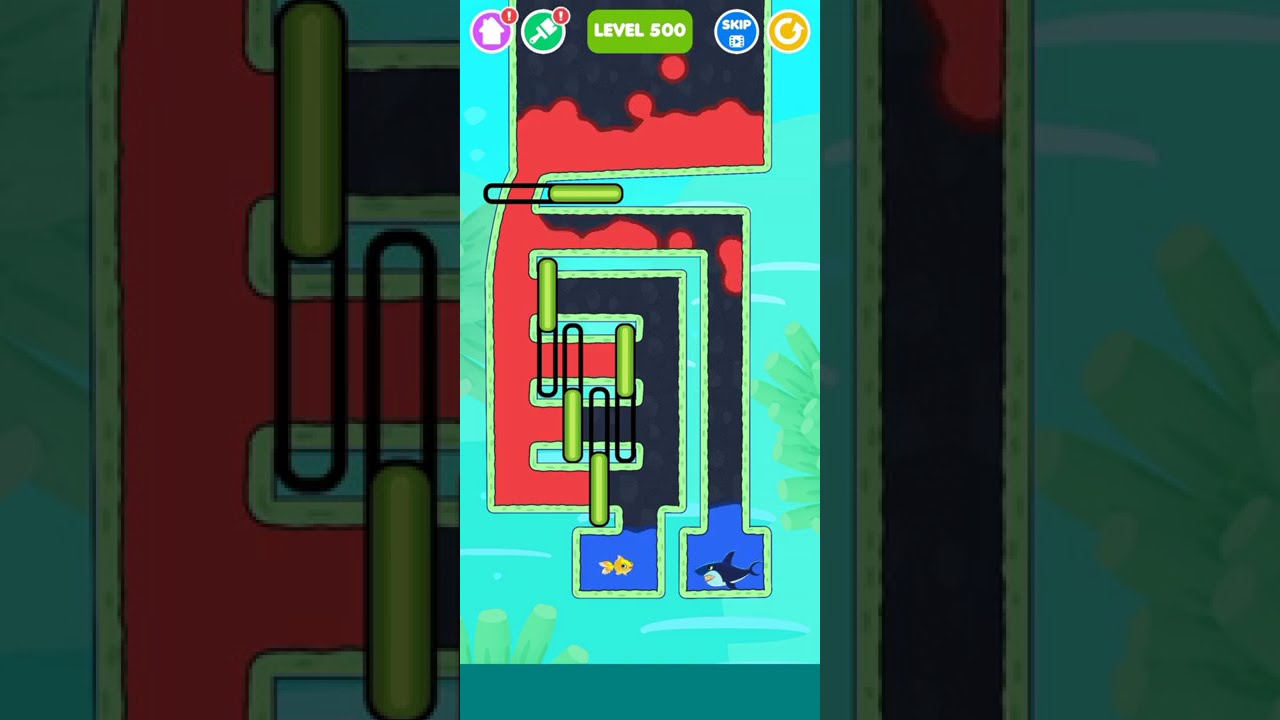The image showcases a vividly colorful and cartoony screen capture of a mobile puzzle game at level 500. The objective of the game appears to involve moving barriers to channel flowing lava from the top of the screen towards a shark located at the bottom. On one side of the game's maze, there is a goldfish, while the other side hosts the shark. The top of the screen features a series of icons, including a home button, a paintbrush button, and a refresh button, with the central text clearly stating 'Level 500' and a 'skip video' option to the right. The overall aesthetic recalls popular mobile game advertisements seen online, emphasizing playful graphics and problem-solving elements that may hint at cognitive skill enhancement.